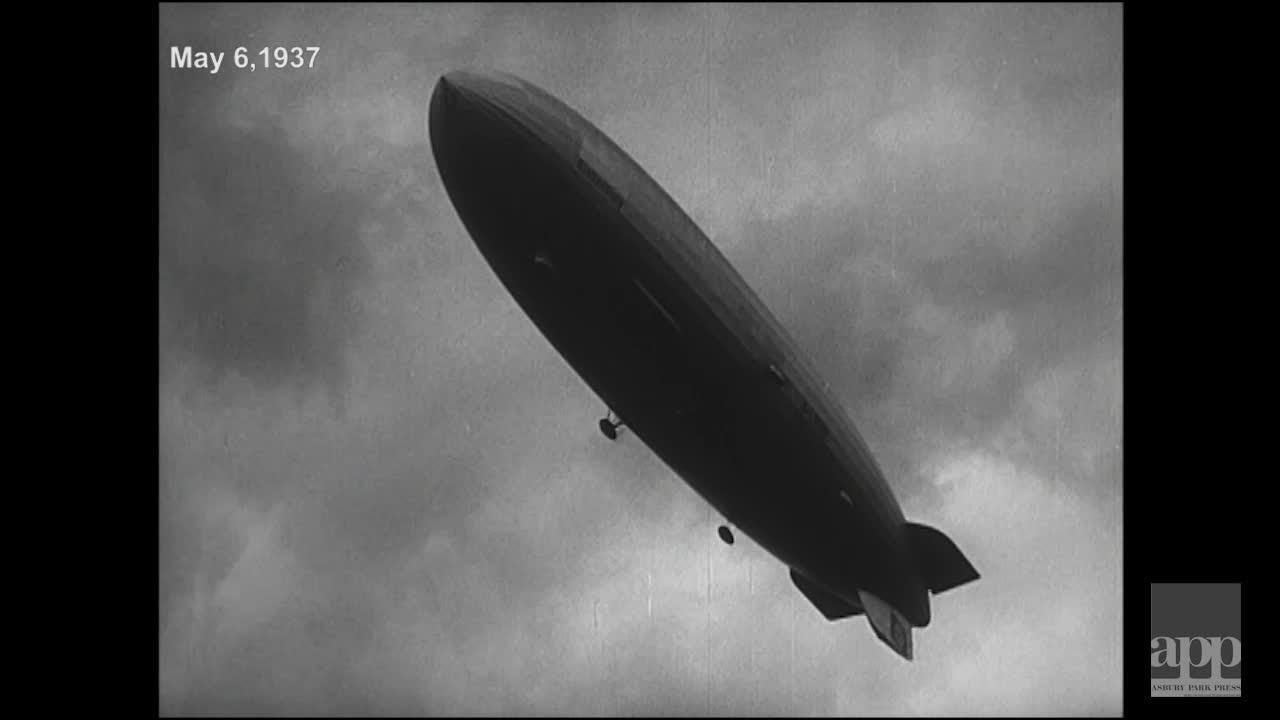This black-and-white photograph, dated May 6, 1937, showcases a large blimp-like airship set against a dark, ominous, and cloudy sky. Captured from a ground view, the massive airborne vehicle features a giant balloon on top and a steel-like torpedo-shaped structure beneath it. Visible from this angle, there are two pods or gondolas attached to the bottom and multiple wheels in the center and towards the front of the airship, possibly landing gear. The back of the airship boasts three propellers—two mounted on the sides and one on the bottom—along with several fins or winged tips. This airship resembles the iconic Hindenburg in design. In the bottom right corner of the photograph, a gray square logo with the text "APP" and some illegible smaller text is visible against a black background, suggesting a museum-like stamp.